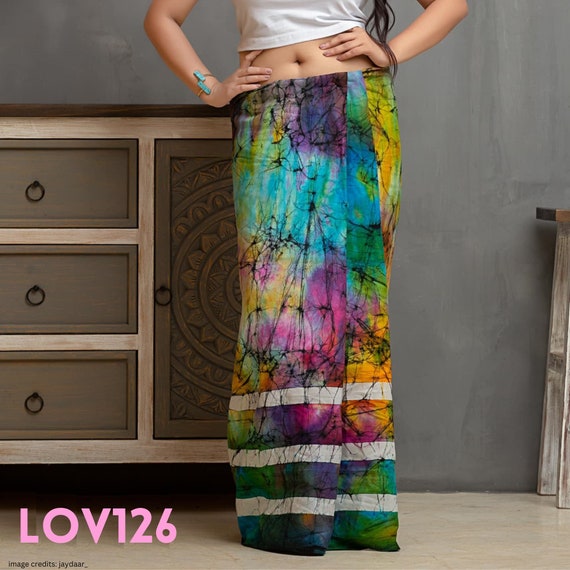The image captures the lower half of a woman or teenager standing in a room with a blended gray wall in the background. The subject is dressed in a white crop top, exposing her navel, and wears a multicolored skirt featuring purple, blue, yellow, green, and thin black lines, with three horizontal white stripes at the bottom. Her hands rest confidently on her hips, adorned with a teal blue rope bracelet on her right wrist, and her long brownish-black hair drapes over her left wrist. She stands in front of a light wood-colored dresser with three circular-handled drawers arranged vertically. The floor appears to be shiny, possibly waxed tile. In the lower left corner of the square image, the text "LOV 126" is displayed in pink, with additional, smaller, unreadable text beneath it.